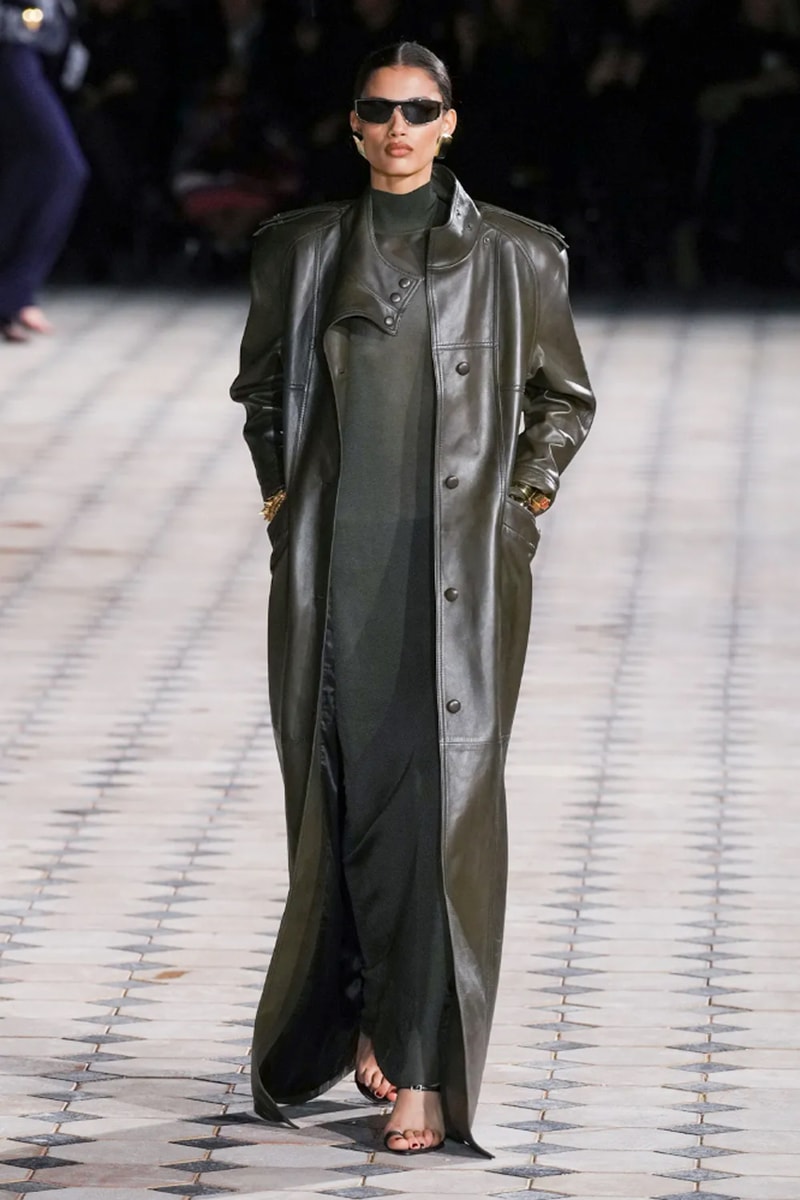This photograph captures a female runway model showcasing a minimalist and somewhat plain outfit. She is dressed in a dark brown leather trench coat that reaches all the way to the floor, with a distinct button detail around the neck area. Underneath, she wears a long, modest black dress with a few buttons. Her footwear consists of sandals with a small heel and a strap across the top of the foot. The model's brown hair is pulled back, and she wears androgynous black sunglasses, enhancing her stern, pouty expression. Her hands are firmly placed in the coat's pockets, adding to her composed demeanor. The runway floor beneath her features a white with black squares pattern, and in the background, a person wearing blue pants is partially visible.